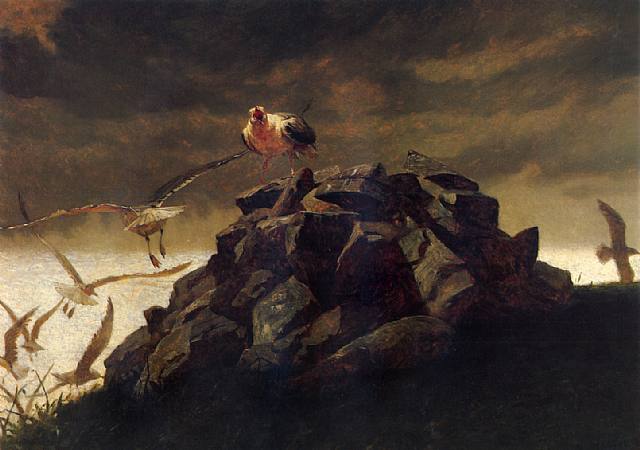This detailed painting vividly captures a dramatic scene featuring several birds against a dark and stormy sky. The sky, with its streaks of brownish gray and yellow, creates a moody atmosphere, appearing darkest in the top left corner. In the foreground stands a large, jagged rock formation, rendered in deep charcoal gray, almost black tones. Atop this rocky mound sits a lone bird, likely a seagull, with a cream-colored body and dark-colored wings, gazing directly at the viewer. Around this central figure, six more birds are depicted in flight, moving in various directions. Some birds soar to the left, over and into a body of white-tinted water, while others head to the right, adding a dynamic sense of movement to the composition. The entire scene is a harmonious blend of nature's raw elements and the birds' animated presence, set against a vividly hued yet ominous backdrop.